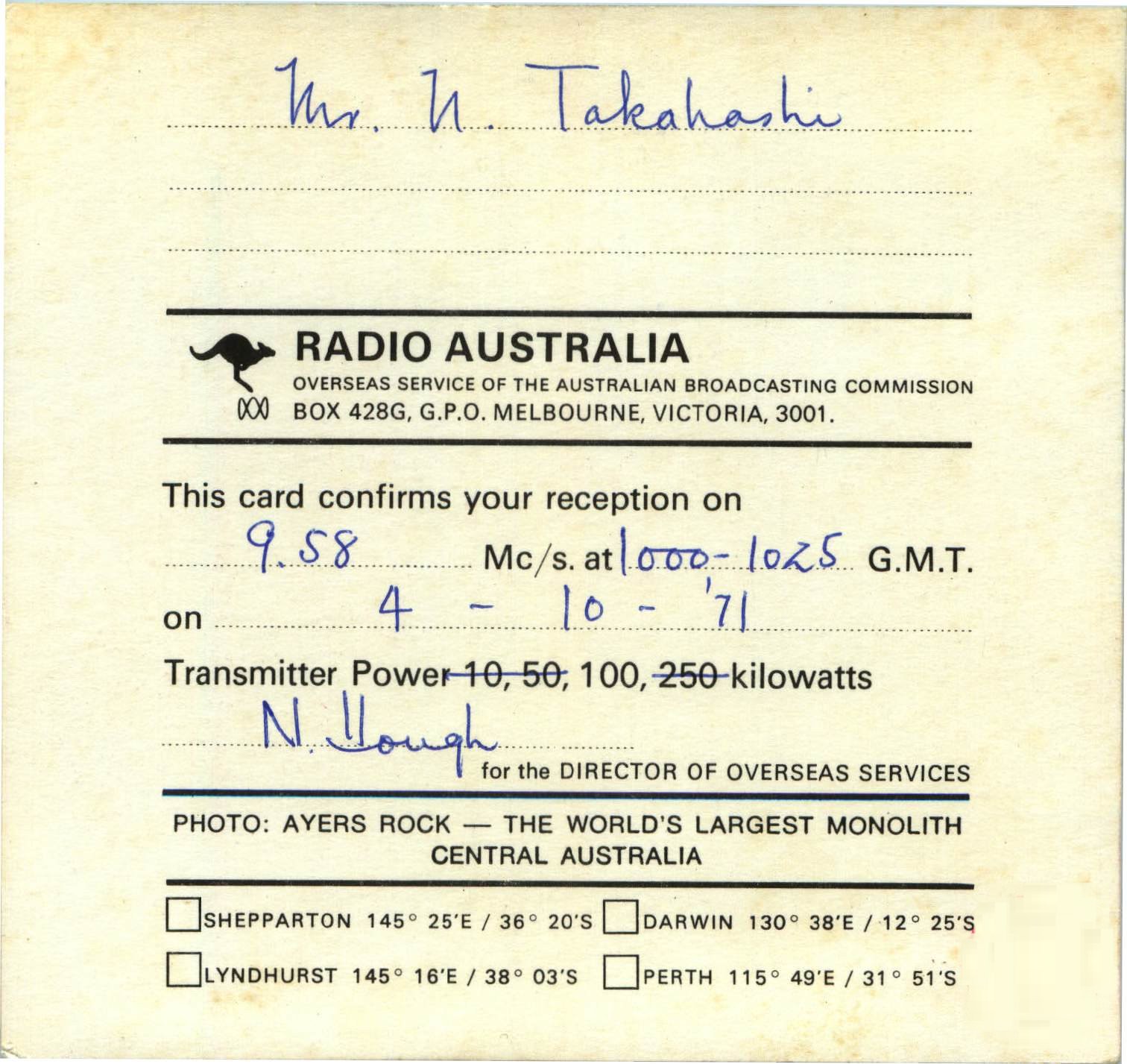This image features an aged, yellowed receipt or certificate, likely due to time. At the top of the light-brown paper, some text is written in green and blue ink, while other parts are in black computer-printed fonts. First, the name "Mr. N. Takahashi" is handwritten at the very top. Following that, there are three dotted lines, with the top one featuring the blue signature.

Beneath the signature and dots, the document displays a black logo for Radio Australia, depicting a filled-in kangaroo facing right. Adjacent to the logo, the text reads: "Radio Australia, Overseas Service of the Australian Broadcasting Commission," along with the address "Box 428G GPO Melbourne Victoria 3001." The card confirms a reception on 9.58 MC-S at 1000-1025 GMT on 4-10-71, specifying a transmitter power of 100 kilowatts. Below, it bears the signature, likely of N. Howe, for the Director of Overseas Services.

Additionally, the card contains a photo captioned "Ayers Rock, the world's largest monolith, Central Australia." Towards the bottom, there are four checkboxes, probably meant to be marked, along with coordinates written nearby, emphasizing further verification details.